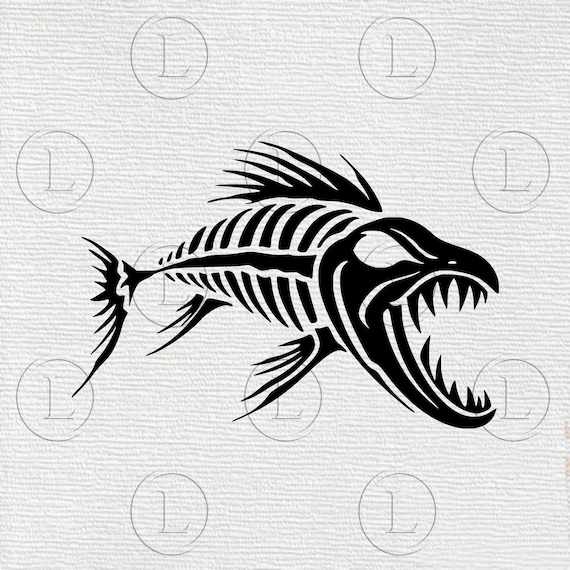The image features a strikingly detailed, black and white tattoo-style artwork of a prehistoric-looking fish skeleton set against a beige, paper towel-textured background. The fish, oriented from left to right, showcases an aggressive appearance with its large, open mouth filled with sharp teeth and its downward-gazing eyes. The head is prominent, and the skeletal body reveals the backbone and ribs, along with multiple spiky dorsal fins and a sharp tail fin. Surrounding the fish are several circular logos with an uppercase 'L' inside them, arranged almost as a pattern across the backdrop, amounting to around ten or eleven circles. The overall design integrates both artistic and graphic elements, evoking a sense of ancient, underwater menace.